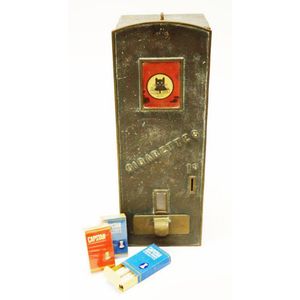The image depicts a vintage metal cigarette dispenser, measuring approximately 12 inches in height, with a dark gray, rusted exterior suggesting considerable age. Central to the box is a red square with a yellow circle inside, featuring the head of a black cat in the middle. Directly below this emblem, the word "Cigarettes" is prominently displayed in a horizontal fashion, with a one-cent coin slot for operating the dispenser. Surrounding the dispenser are various small, vintage cigarette packs, some visibly aged and worn. Notably, there are two blue packs positioned at the bottom, a red pack on the left side, and another blue container near the machine. The overall design and condition of the object emphasize its historical nature and purpose as an old-fashioned cigarette vending machine.